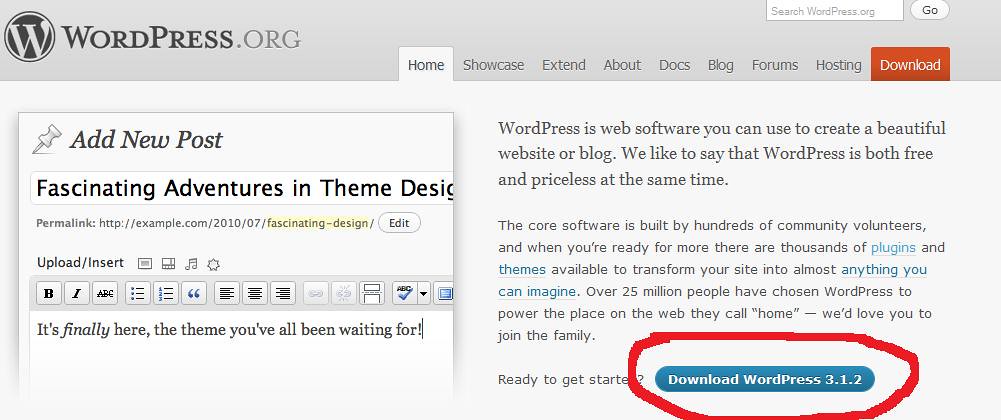The image is a rectangular screenshot from a computer, showcasing a webpage from WordPress.org. The header, spanning the full width at the top, is gray and contains a black circle with a light-colored "W" on the left, next to "WordPress.org" in black text. On the far right of the header, there is a white search box labeled "Search WordPress.org" with a "Go" button beside it. Centrally, the header features several tabs: Home (which is currently open), Showcase, Extend, About, Docs, Blog, Forums, Hosting, and an orange rectangle with the word "Download" inside.

The main section of the page below the header is divided into two parts with a light gray background. On the left side, there is a section for adding a new post, titled "Fascinating Adventures in Theme Design." It includes a permalink displayed as "http://example.com/2010/07/fascinating-design/edit." Below this, there are options to "Upload Insert" media, and a toolbar with various formatting buttons for bold, italic, font changes, spacing adjustments, quotations, and text alignment. The initial post content reads, "It's Finally Here, the theme you've all been waiting for."

On the right half, the page describes WordPress: "WordPress is a web software you can use to create a beautiful website or blog. We like to say that WordPress is both free and priceless at the same time. The core software is built by hundreds of community volunteers, and when you're ready for more, there are thousands of plugins and themes available to transform your site into almost anything you can imagine." This section concludes with a call to action, "Over 25 million people have chosen WordPress to power the place on the web they call home. We’d love you to join the family. Ready to get started?" followed by a blue oval button with white text, "Download WordPress 3.1.2," highlighted with a red oval.

The cohesive layout, combined with the clear prompts and informative content, effectively introduces users to WordPress and encourages them to begin using the platform.